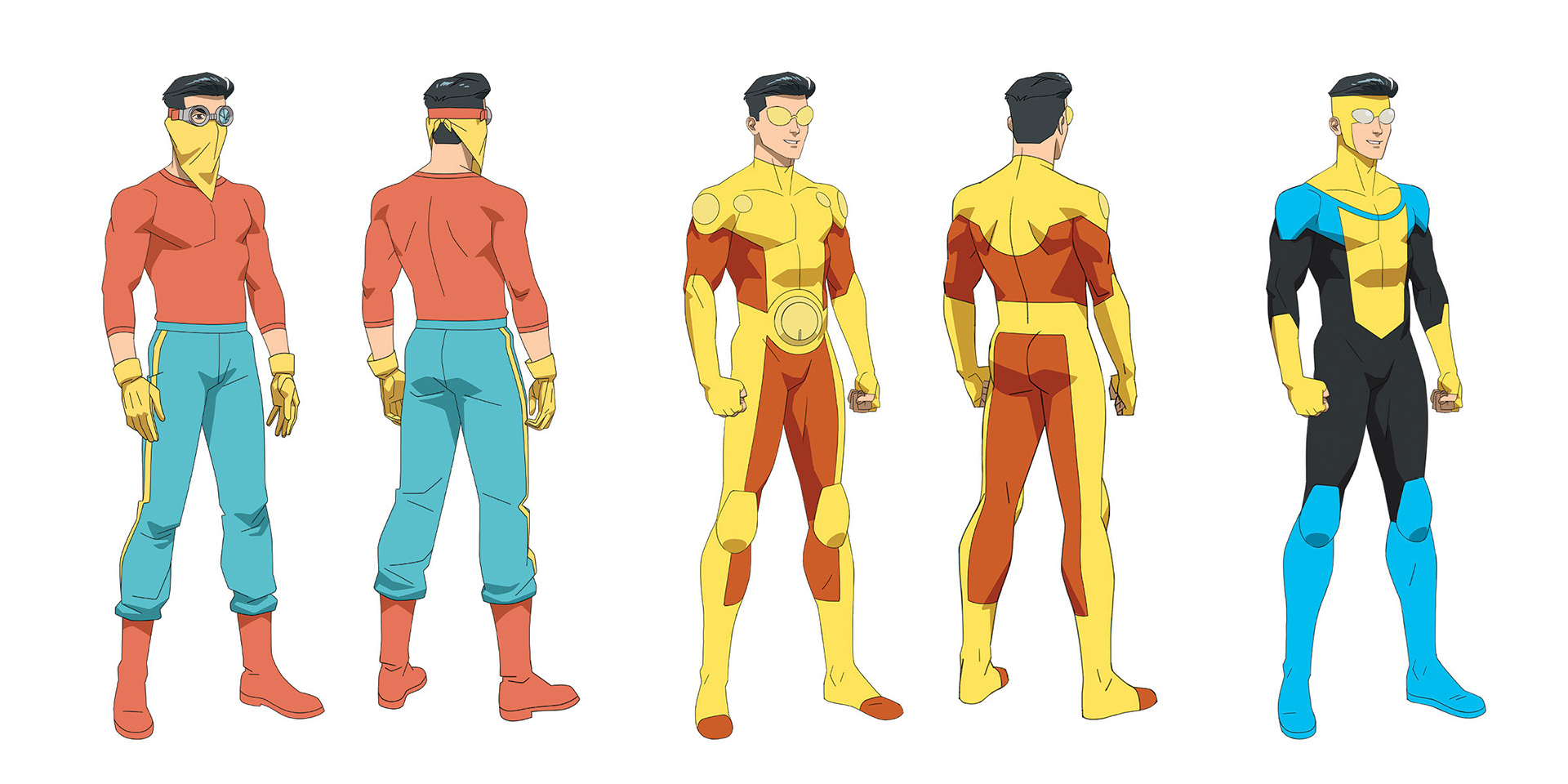The image showcases five illustrations of the same superhero character in various outfits, presented from different angles. Starting from the left, the character is depicted in a salmon shirt, blue pants, and blue boots, with a yellow bandana covering his face and goggles on; one view is front-facing, and the other is from the back. The next set of illustrations features the character in a yellow and red armored suit with matching yellow glasses, again showing both the front and back perspectives. The final depiction shows the character in a blue, yellow, and dark blue costume, this time only from the front. In this outfit, the mask covers his face, revealing his mouth. The consistency across the different depictions emphasizes the dynamic nature of the character's appearance.